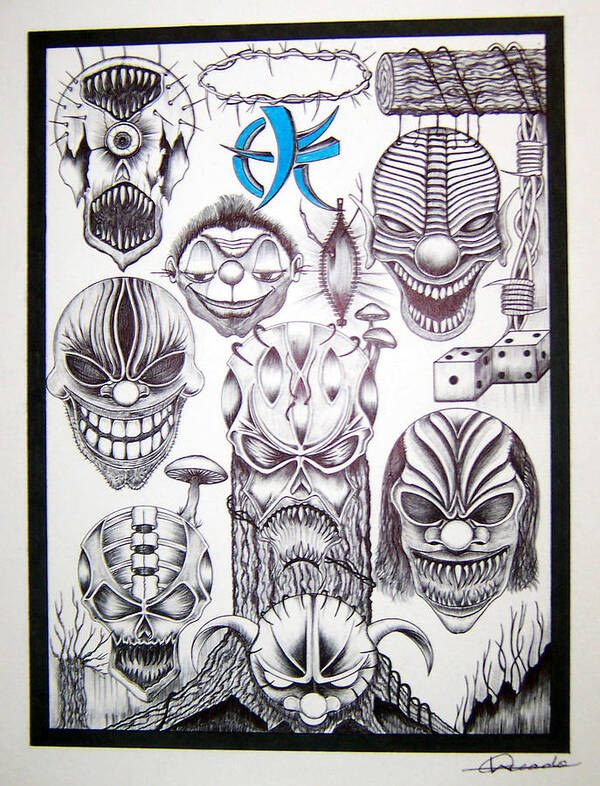The image appears to be a hand-drawn, illustrated poster on a cream-colored or off-white background, framed by a black border. The central elements of the poster are a collection of seven to eight menacing masks and monstrous faces, rendered in black ink with a charcoal-like texture. These masks are diverse in their frightening characteristics: one resembles a skull, another features sharp horns, while one has the terrifying visage of a fanged clown. Additional disturbing details include a face with nails sticking out, a cyclops with a mouth on its forehead filled with sharp teeth, contributing to the overall eerie tone.

At the bottom of the poster, intricate root patterns are depicted, adding to the unsettling atmosphere. The upper right corner features a log wrapped in barbed wire with dangling dice on a cord, while a mushroom also appears among these chaotic elements. The top center of the poster is uniquely highlighted with stylized initials, vividly colored in blue, which appear to be 'E' and 'K'. In the bottom right corner, there is a signature rendered in black, marking the artist's presence.